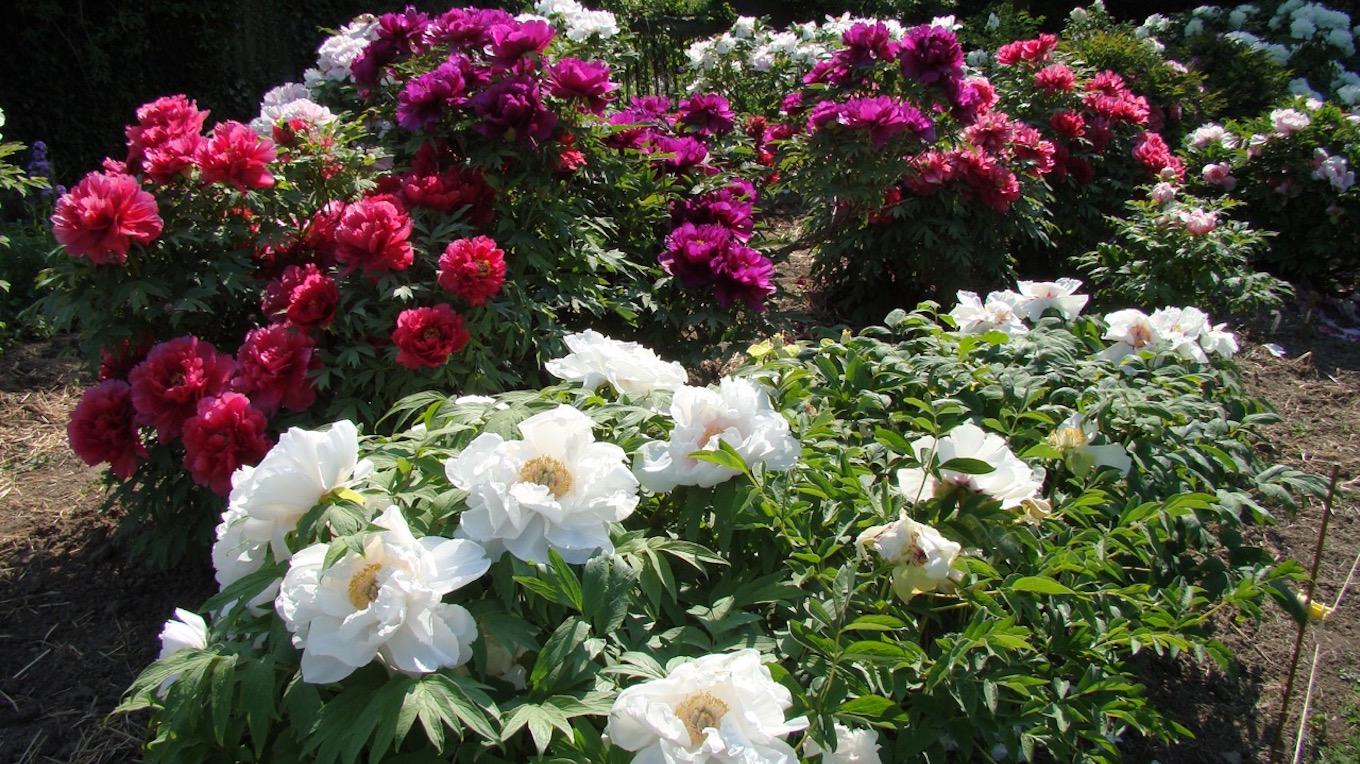This vibrant daytime photograph of a meticulously maintained flower garden showcases an array of blooming flowers in vivid detail. The garden features rows of flowers, each of different colors, with dirt pathways in between for easy access. In the foreground, clusters of white flowers with yellow centers, resembling daisies, stand out. To the left, pinkish-red flowers, possibly carnations, and smaller bluish ones at the far top left, add to the diverse palette. As the eye moves further back, there are bursts of orange and purple flowers, creating a magnificent tapestry of colors.

The leaves are a lively green, indicating the health and care given to the garden. A small metal pole with a wire fence on the right suggests efforts to protect the plants from animals. The sunlit scene emphasizes the bright, varied hues of the flora against the clear brown dirt, free of weeds. This beautifully bloomed garden, enhanced by a vivid array of white, orange, pink, magenta, and purple flowers, exemplifies the gardener's skill and dedication.